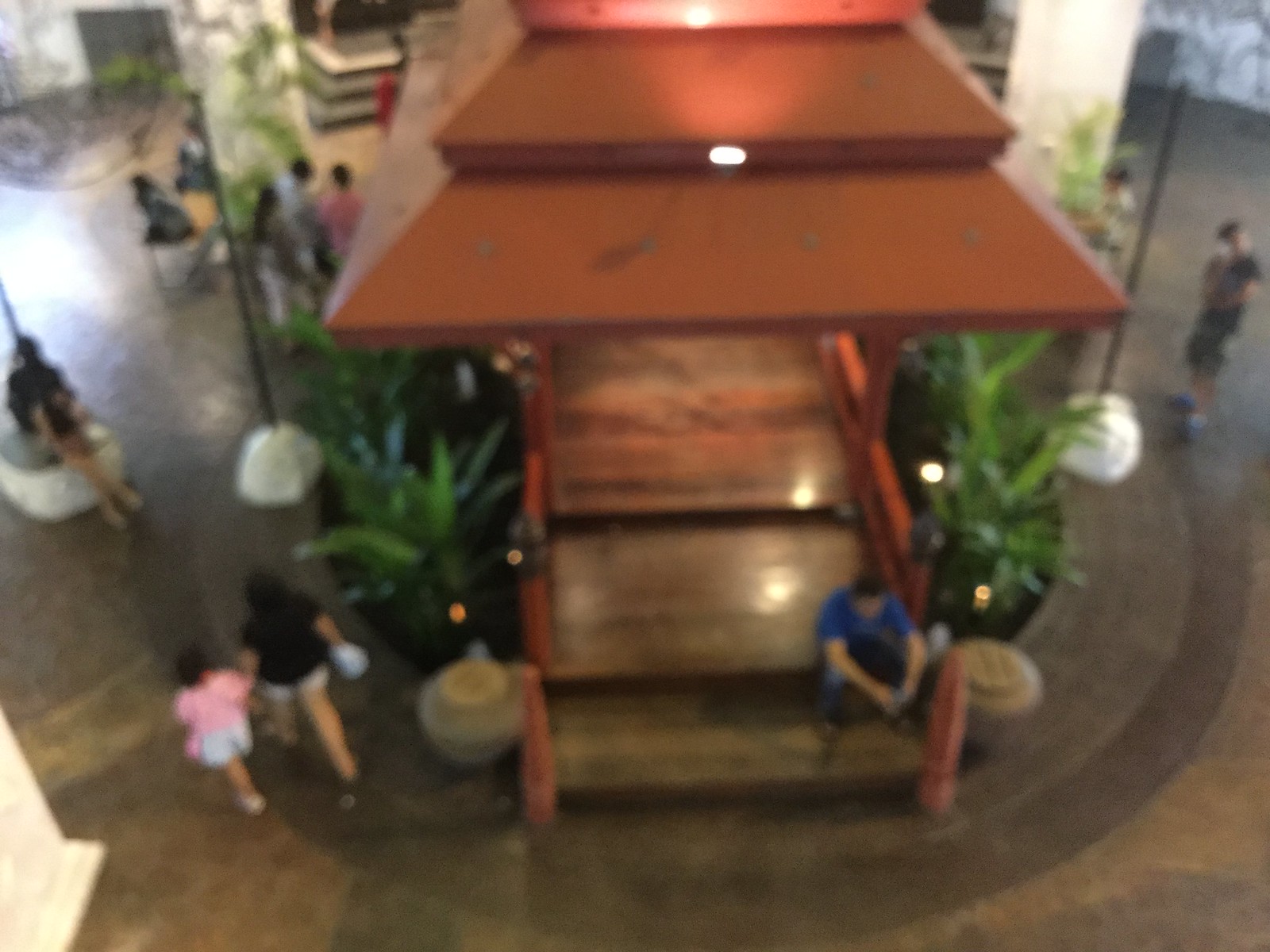An aerial photograph captures the bustling lobby of a large indoor space, centered around a striking pagoda-style structure with a vibrant red tiered roof. A man with dark hair, wearing a blue short-sleeved shirt and dark pants, sits on mid-brown toned steps beneath the pagoda, surrounded by lush green plants and encircled by a red railing. Below, the floor is a blend of tan and brown hues, contributing to the earthy ambiance.

To the side, a woman with dark hair, dressed in a black shirt and white shorts, stands with her young daughter, who is clad in pink and white attire. Various other individuals meander through the scene, contributing to the lively atmosphere. The space also features roped-off sections and strategically placed black metal poles, adding structure and organization to the area. In the background, elegant white columns stand tall, enhancing the lobby's grand and open feel.